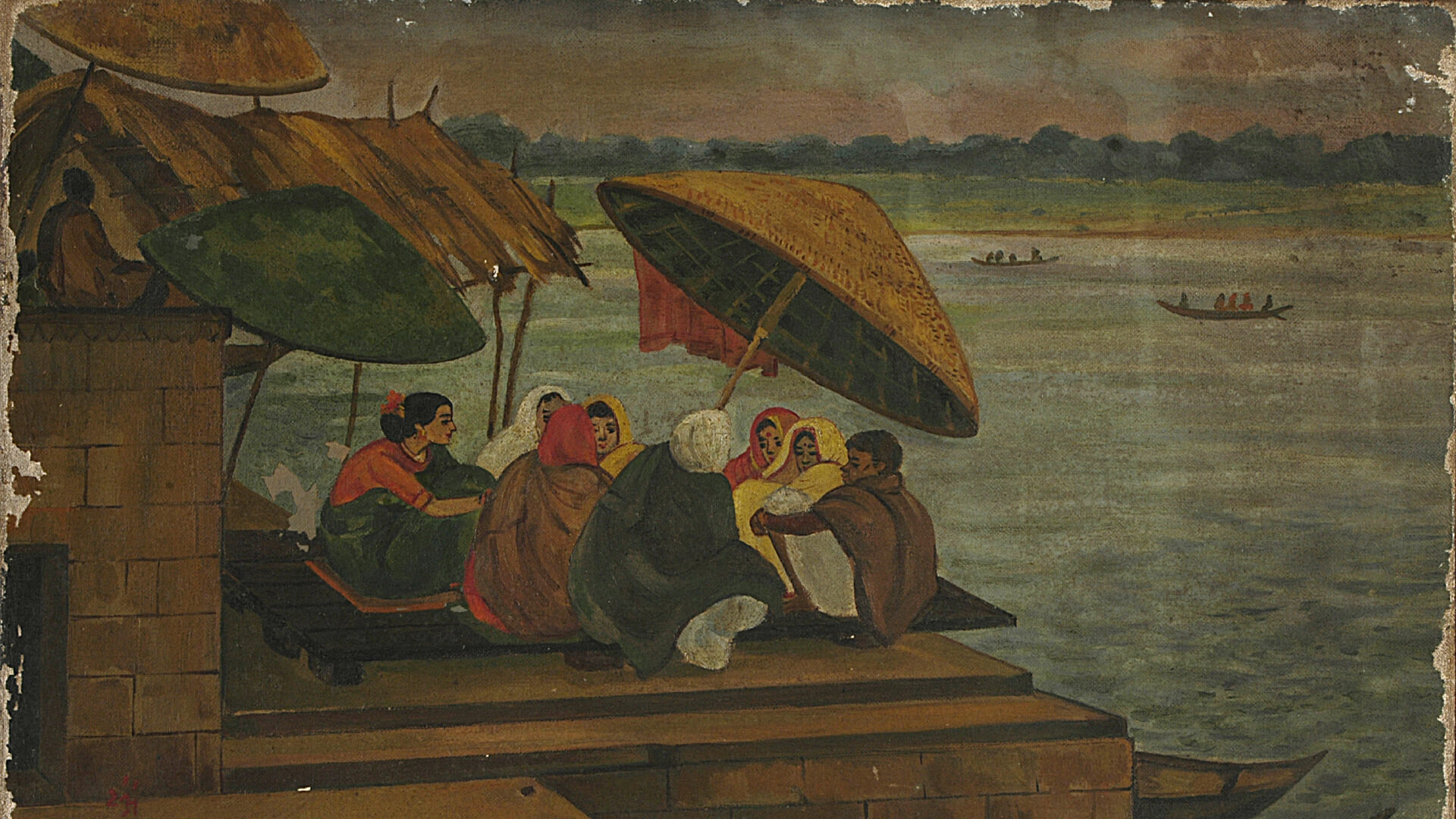The image is a photograph of artwork that appears to be created in a modified Japanese or Chinese style, possibly using pastel. The painting is dark and muted, possibly dirty or aged, with worn sections and chipping around the edges. It depicts a small group of brown-skinned people, dressed in loose robes and hoods, sitting in a circle on a wooden platform over a stone flat surface by the edge of a lake. They are shaded by three umbrellas—two yellow and one green—with one yellow umbrella adorned with a piece of red fabric or flag. One woman is seated on a pad. A straw-roofed structure is partially visible behind them to the left. The lake in the background features two canoes, each carrying three to four people, and beyond the water lies a landscape of grasslands, bushes, and indistinct mountains or trees, under a dark gray and red sky.